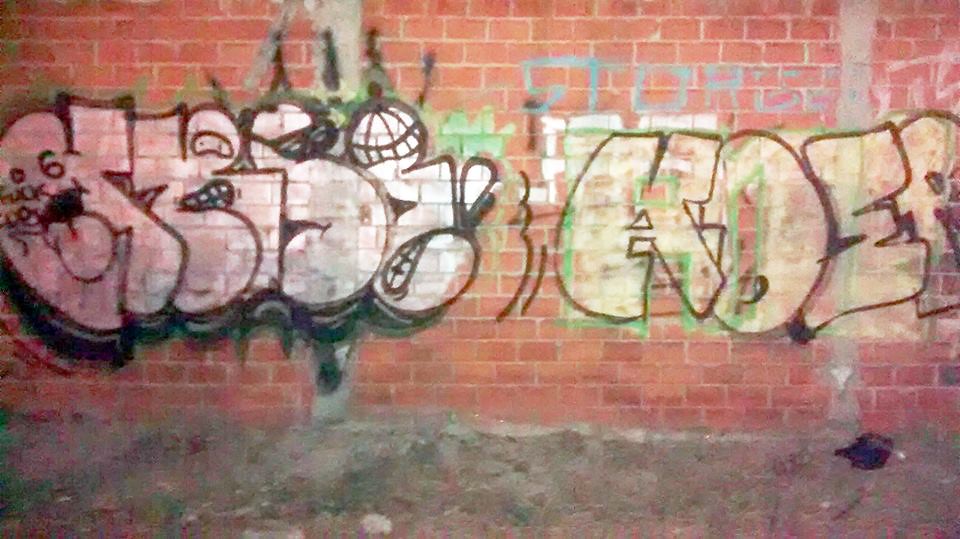The image features a close-up of an old, orange-colored brick wall covered in multiple layers of colorful graffiti. The wall appears dirty and grimy, especially near the bottom, which may either be due to dirt accumulation or a visually indistinct concrete base. The graffiti includes various letters and words, though not all are fully readable.

There are several notable details:
- **White Graffiti:** Features little faces drawn within the letters and some obscenities, with black borders.
- **Green Graffiti:** Positioned over some white letters.
- **Blue Graffiti:** Letters appear above other layers.
- **Pink Graffiti on the Left:** Possibly says "greasy" or "grease," outlined in black with a band-aid and a mouth forming part of the design. This mouth is white and black, with a tongue outlined in black.
- **Black Lettering:** Includes a prominent number six, "F-U-X," and something resembling "goo" or "coo." There is a crown and a world outline in black on the left.
- **Yellow Graffiti:** Appears to spell a word like "ater," outlined in black with green filling.
- **Blue Graffiti:** Includes what seems to be the word "story."
  
Additionally, mentions of white lines above some of the graffiti letters and a piece of cloth material on the ground, which appears blue and white, are observed. There are no people or objects other than the graffiti and wall visible in the photo.